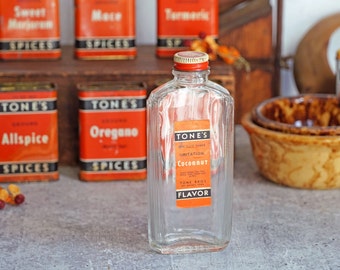The photograph showcases a collection of vintage Tones spice containers, predominantly featuring a clear glass bottle in the foreground. This bottle, presumed to be of coconut flavor, has a striking orange label adorned with white text. The brand's name, Tones, is displayed prominently on a blue banner at the top of the label. The word "flavor" is inscribed at the bottom of the label, also in white text on a dark blue banner. This central bottle appears empty.

In the background, there are five Tones spice containers, each with unique spices including oregano, allspice, sweet marjoram, maize, and turmeric. The containers are a vibrant orange with dark blue or black accents and white text, lending a vintage charm to the ensemble. Additionally, to the right of the image, there's a light brown and yellow bowl with some contents, all set on a gray or granite-style countertop. The arrangement of these items, combined with the clear focus on the bottle in the foreground, creates a nostalgic and detailed depiction of culinary essentials.